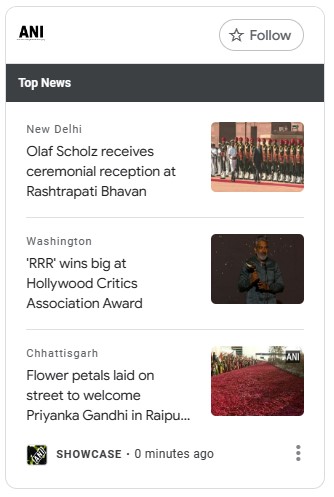Screenshot of a mobile app displaying top news stories. 

At the top, the title "ANI" is located in the upper left corner and a "Follow" button with an unchecked star icon is in the upper right corner. Below this, a navigation bar labeled "Top News" spans horizontally. 

The first news story is from New Delhi: "Olaf Scholz receives a ceremonial reception at Rashtrapati Bhavan," accompanied by an image of several soldiers in formal attire. 

The second headline comes from Washington: "RRR wins big at Hollywood Critics Association Award," alongside a picture resembling the iconic "Most Interesting Man in the World."

Further down, another story reads: "Flower petals laid on the street to welcome," with an image displaying a path strewn with vibrant flower petals. 

The app indicates this content was updated "0 minutes ago," and features an ellipsis for additional menu options.